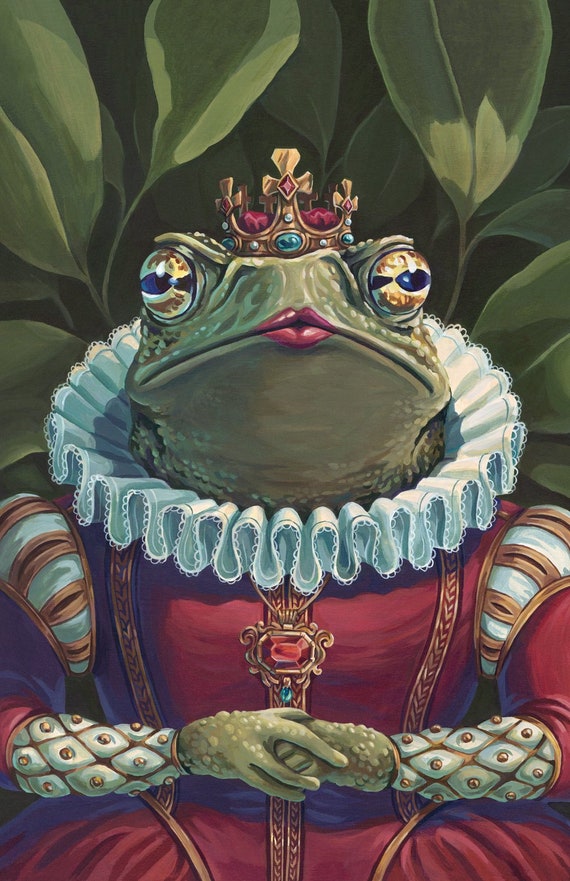The digital artwork depicts a cartoon frog adorned in regal attire, sitting serenely in front of a fan-shaped array of large, dark and light green leaves. The frog wears a golden crown embellished with red jewels and has striking red lipstick, potentially indicating it is a princess. The frog is dressed in an elaborate outfit featuring a ruffled collar that encircles its neck, a tight-fitting bodice with capped sleeves, and a flowing dress cinched at the waist. Additionally, it sports a red ruby necklace that complements the crown. The frog's hands are gracefully folded in front of it, adding to its royal demeanor. The color palette of the image includes vibrant greens, reds, blues, golds, yellows, oranges, and maroons, enhancing the detailed and whimsical nature of the scene.